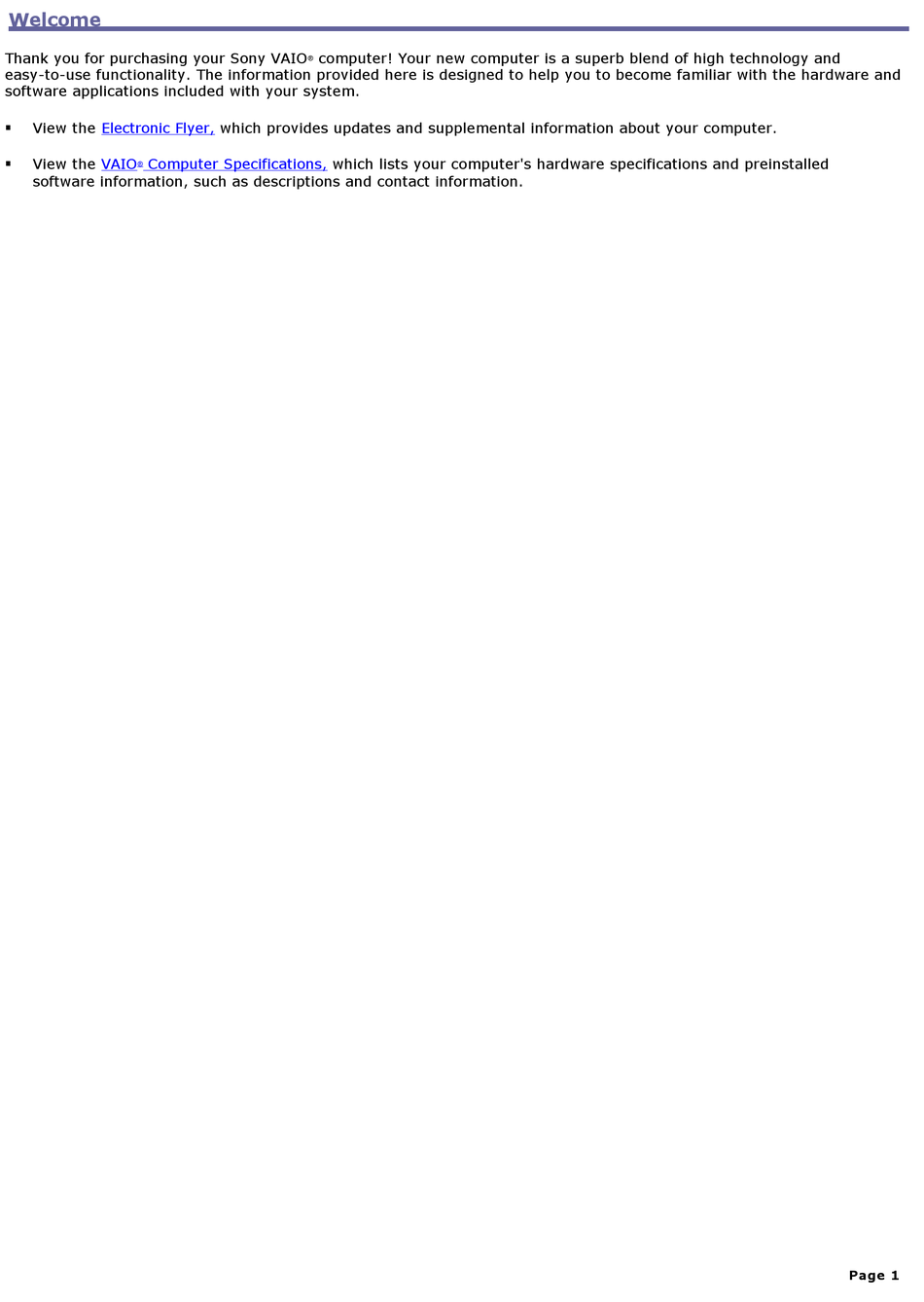This image is a screenshot of what appears to be a digital manual or purchase confirmation page, possibly for a Sony VAIO computer. The page features a predominantly white background. The top of the page displays the word "Welcome" in blue text, followed by a long blue line that serves as a section divider. Below this, a block of black text expresses appreciation for the user's purchase. It reads: "Thank you for purchasing your Sony VAIO computer. Your new computer is a superb blend of high technology and easy-to-use functionality. The information provided here is designed to help you to become familiar with the hardware and software applications included with your system."

The text continues with two bullet points. The first bullet point instructs users to "view the electronic flyer," where "electronic flyer" is a blue hyperlink. This flyer is said to provide updates and supplemental information about the computer. The second bullet point advises users to "view the VAIO computer specifications," with "VAIO computer specifications" also being a blue hyperlink. This section lists the computer's hardware specifications and pre-installed software information, including descriptions and contact information. The bottom of the page is simply white space, with no additional images or figures, reinforcing the minimalist design. The footer indicates that this is page one of the document.